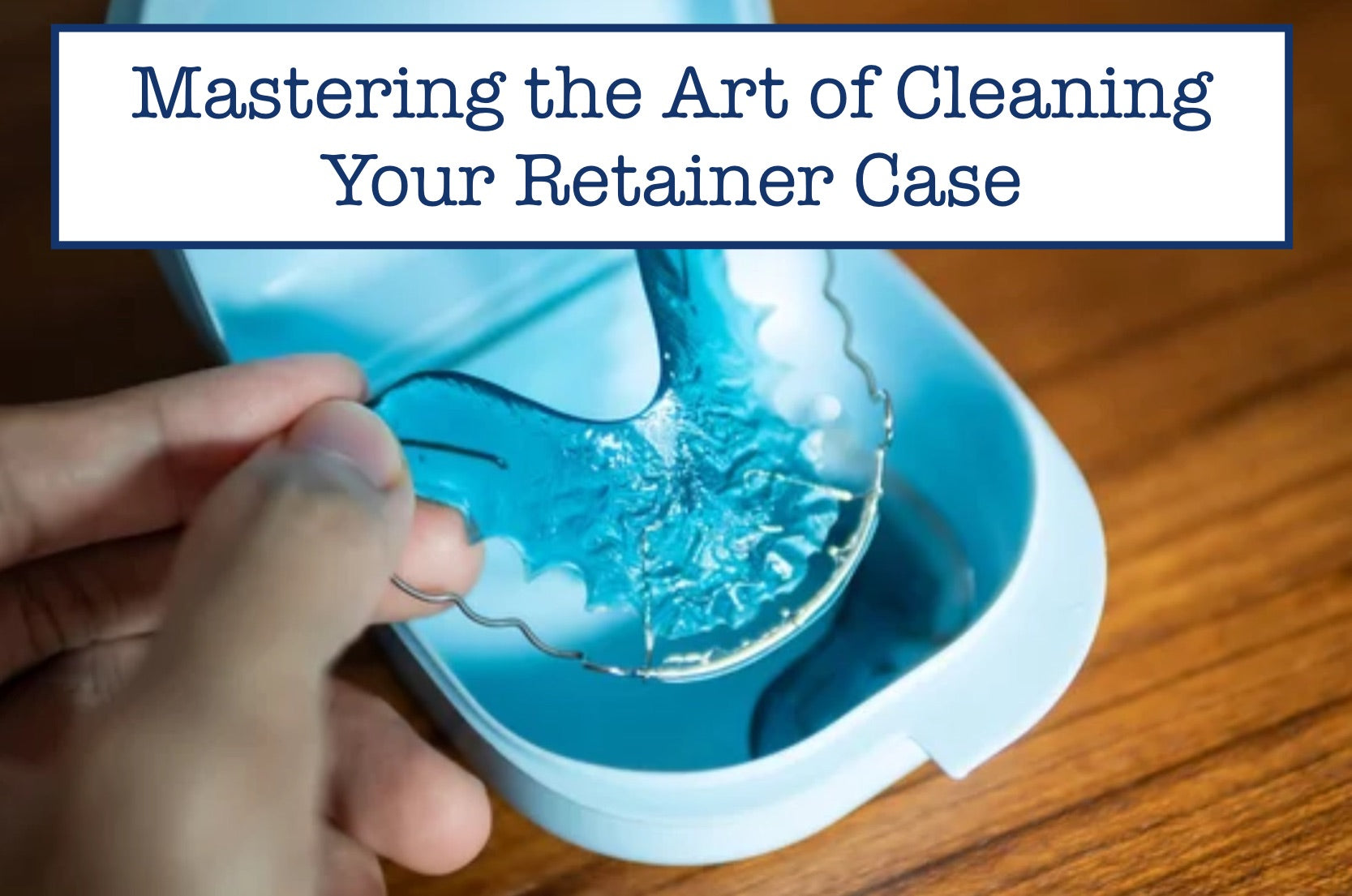This professional, instructional photograph, potentially part of a brochure, is centered around the theme "Mastering the Art of Cleaning Your Retainer Case," displayed in blue text on a white background at the top of the image. The scene captures a left hand, possibly belonging to a preteen with slightly brown skin, holding a moist, translucent retainer molded to fit the upper teeth. The retainer is designed with a wire and shows clear imprints of the palate. It is positioned above a blue and white retainer case, which rests open on a wood grain surface. The angle of the shot is from above, offering a close-up view that emphasizes the detailed, professional quality of the photograph.